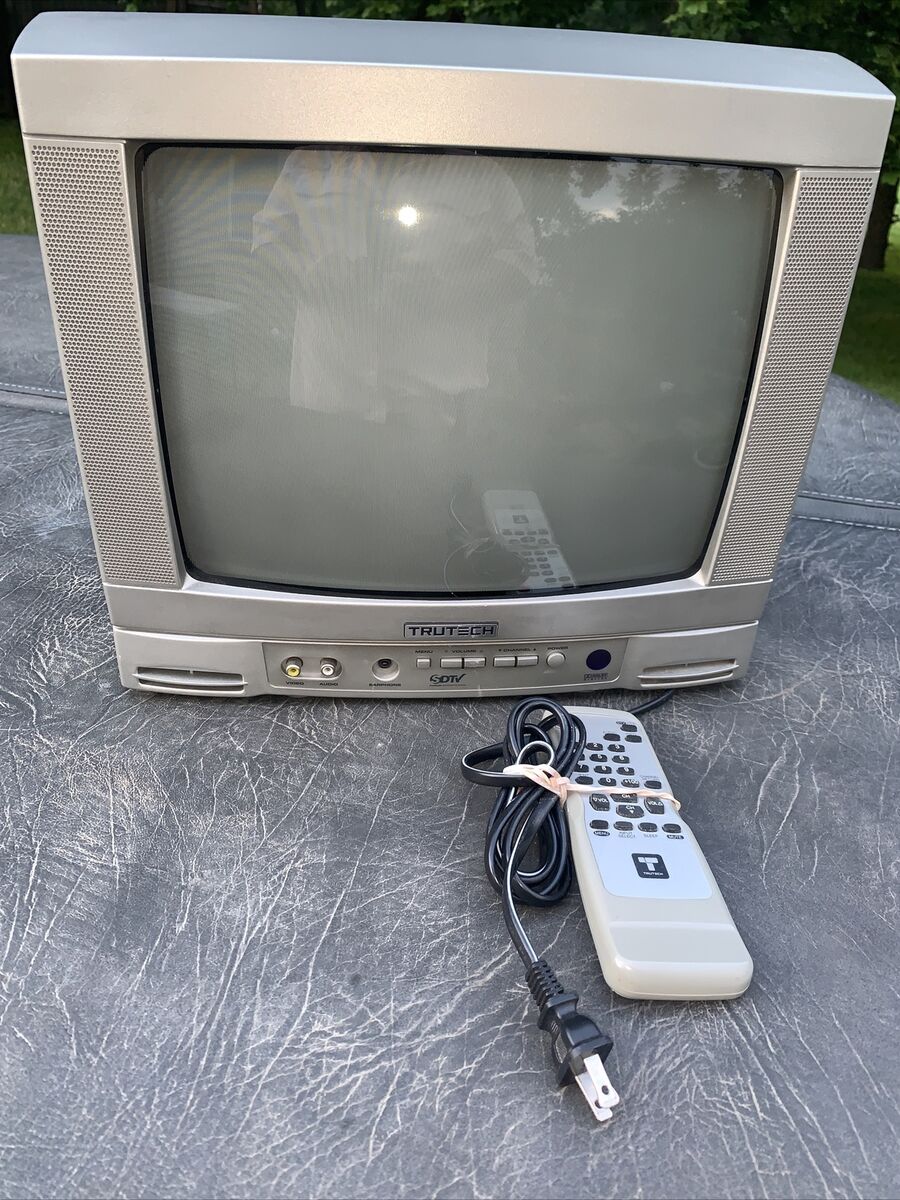This close-up image captures an old tube-style TrueTech television sitting on a cracked and line-marked gray floor, likely concrete. The screen, which reflects a person wearing a white t-shirt and trees in the background, hints at its glossy surface. In front of the TV lies its remote, which is silver at the top with black buttons and a 'T' logo beneath them. The remote, light gray overall, is secured with a rubber band around the center, also holding the power cord. This cord is black with a white stripe and has silver prongs.

The TV’s silver frame includes built-in speakers on the left and right, along with two smaller speakers at the base featuring vent holes. Below the screen, "TRUTECH" is elegantly engraved on a silver plaque. The front panel also presents dual audio-visual jacks: yellow for video input and white for audio input. Moreover, there's an ambiguous small black prong whose label is unreadable. The control panel includes five buttons beneath the plaque, with labels for power, volume, channel, and menu functions, along with an "SDTV" mark in blue. A circular power button and an RF reader, depicted as a small black circle, are also part of the TV’s interface. The image likely serves to illustrate the television's condition, potentially for a marketplace listing.